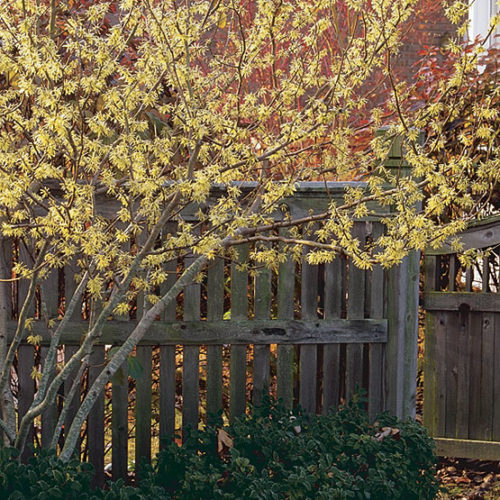In this detailed outdoor autumn scene, a tall wooden fence, approximately six feet high, serves as the backdrop. A prominent, leggy tree with slender, yellow-leafed branches occupies the left half of the image, stretching upwards and dominating the upper portion. Nestled in front of this tree are several green bushes, contributing to the layered composition. Centrally in the bottom part of the image, a partially open wooden gate, part of the fence, hints at recent passage and reveals a bit of the yard beyond. Scattered on the ground are old, brown leaves, emphasizing the autumn setting. Behind the main tree, the reddish foliage of another larger tree adds a vibrant contrast, weaving an intricate blend of seasonal colors throughout the scene.